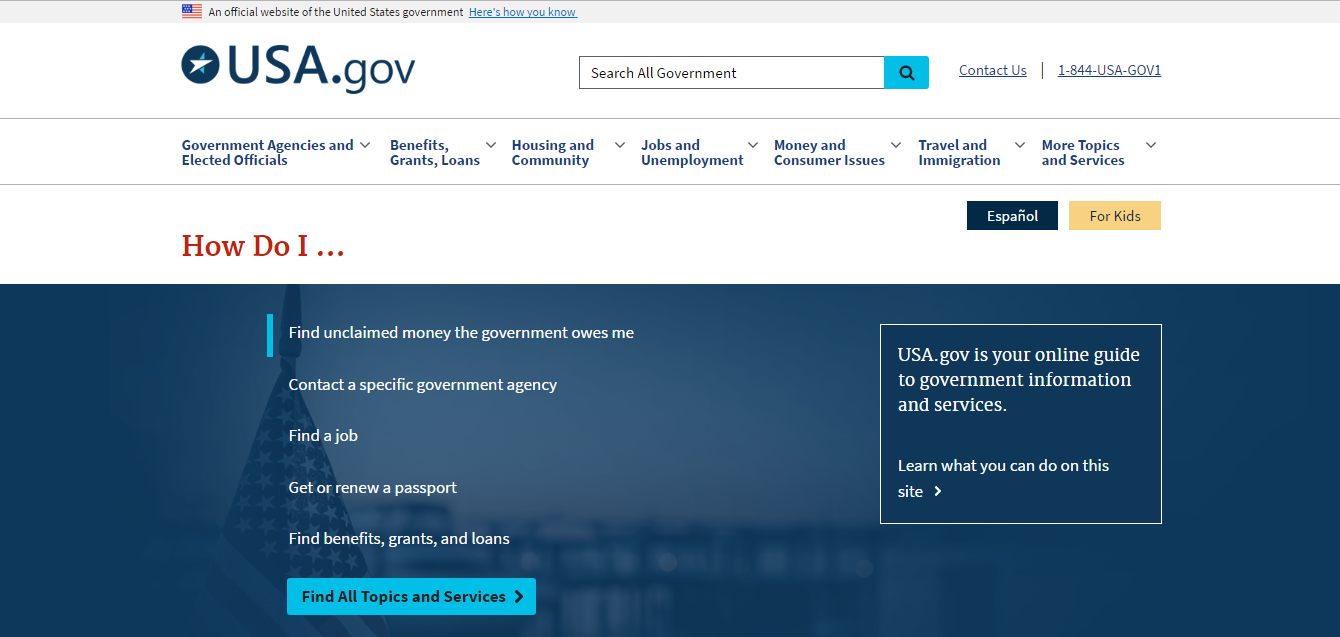This image is a screen capture of the USA.gov website displaying a clean and organized interface. 

At the very top, there's a thin, small banner featuring a small image of the American flag and some hard-to-read gray text. Directly below this, set against a white background, the site prominently displays "USA.gov" alongside a blue icon containing a white star.

Beneath the logo is a comprehensive search bar labeled "Search all government," accompanied by a magnifying glass icon and a blue search button. To the right, blue hyperlinks include "Contact Us" and the phone number "1-844-USA-GOV1."

Following this, several blue-text links serve as dropdown menus for various categories: “Government Agencies and Elected Officials,” “Benefits, Grants, Loans,” “Housing and Community,” “Jobs and Unemployment,” “Money and Consumer Issues,” “Travel and Immigration,” and “More Topics and Services.” 

Further down, the phrase “How do I...” appears in orange text, next to blue and yellowish buttons labeled “Español” and “For Kids,” respectively.

On a blue background beneath this section, white text provides quick links to services: “Find unclaimed money the government owes me,” “Contact a specific government agency,” “Find a job,” “Get or renew a passport,” and “Find benefits, grants, and loans.” Closing this section, a prominent blue button offers access to "Find All Topics and Services."